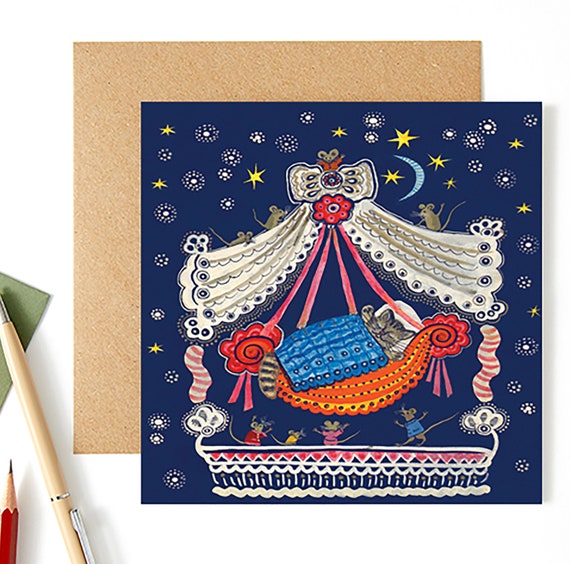This detailed handmade card features a striking illustration set against a navy blue background reminiscent of a nighttime sky, adorned with white and yellow stars alongside small white dots that look like twinkling snowflakes. The focal point of the artwork is a beautifully ornate cradle with an orange and pink curved bed, tied up with pink ribbons and a white lacy canopy topped with a bow and flower. Inside the cradle, a brown kitten sleeps peacefully under a cozy blue blanket. Beneath the cradle, four cheerful mice in red, yellow, pink, and blue outfits look up in admiration. The card, which could be for congratulating a new mother, sits atop a tan square piece of cardboard or paper, matching the size of the card itself. To the left of this arrangement, a pen and a pencil are thoughtfully placed, enhancing the handcrafted charm of this greeting card.